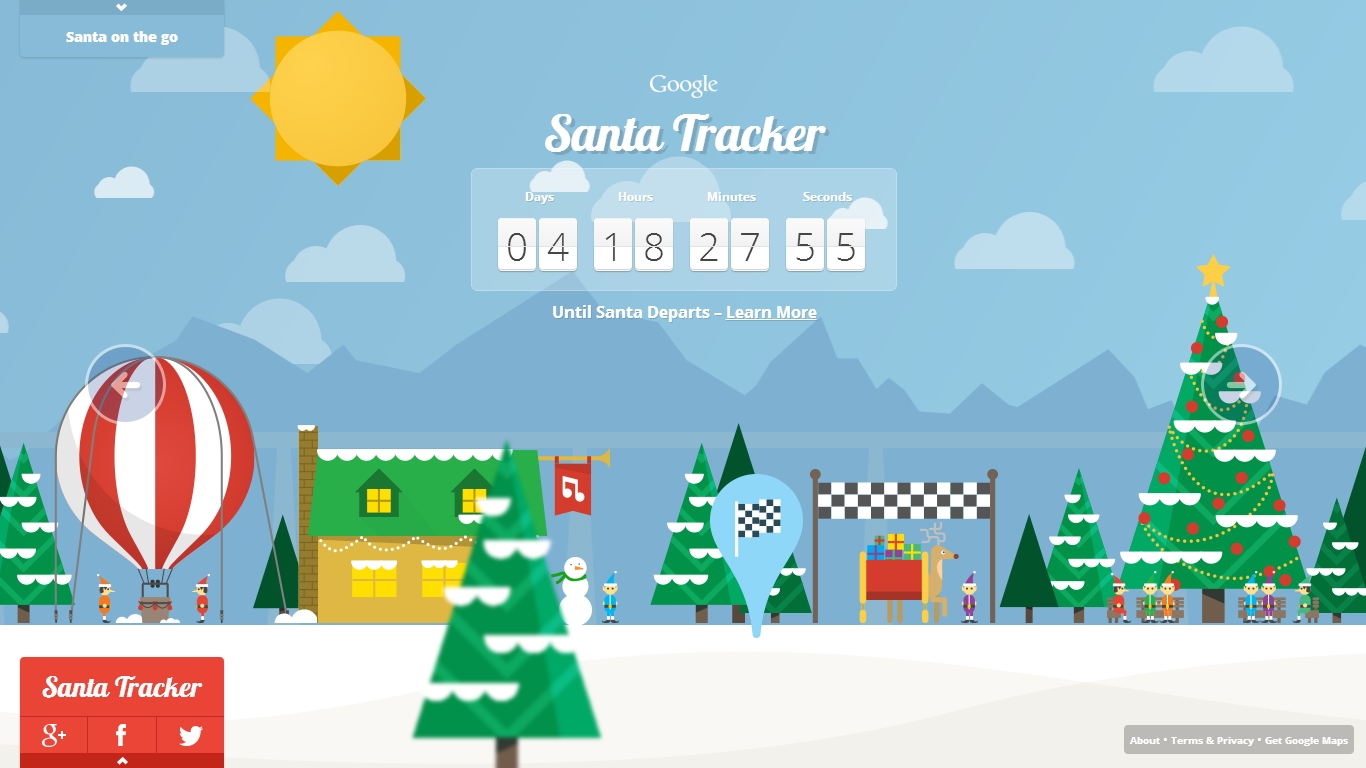This is a vibrant screenshot from Google's Santa Tracker, showcasing a festive countdown until Santa's departure. The central focus displays a countdown timer with "4 days, 18 hours, 27 minutes, and 55 seconds" remaining. The webpage background is adorned with a charming Christmas scene in an infographic style, not photorealistic, but more whimsical and illustrative.

In the backdrop, a serene mountain range stretches under a light blue sky with soft, transparent white clouds. Central to the image is a large peppermint-striped hot air balloon tethered to the ground with two cheerful elves standing next to it. The festive environment is dotted with snow-covered Christmas trees, each illustrated with triangular precision, and a quaint house with a green roof and a chimney nestled among the trees.

On the far right side, a decorated Christmas tree stands tall, gleaming with red ornaments and crowned with a radiant yellow star. Surrounding this tree are six lively elves, adding to the scene's holiday cheer. Adding a touch of excitement, a black and white checkered race banner spans above a reindeer hitched to a classic red sleigh, ready for Santa's journey.

In summary, this visually appealing infographic from Google’s Santa Tracker encapsulates the anticipation and joy of the holiday season with its detailed, picturesque elements and playful design.